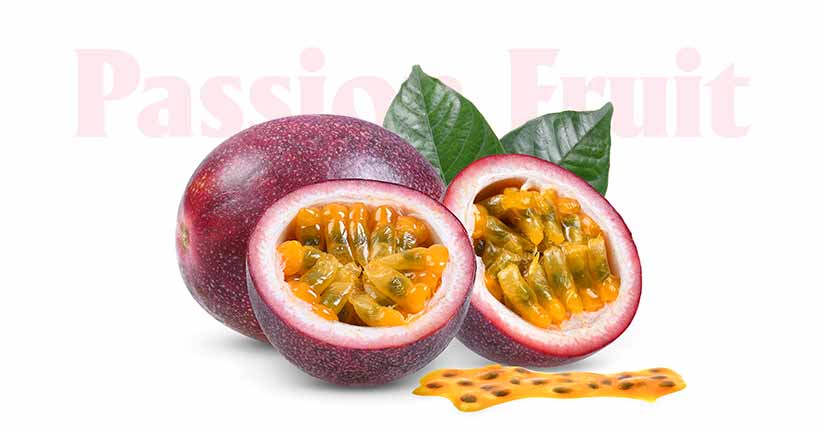The rectangular image, approximately six inches wide and four inches tall, beautifully showcases two pieces of passion fruit against a very pale blue, almost white, background. The whole passion fruit, a red oblong object with little white specks, is positioned in the background to the left, accompanied by two thick, waxy, green leaves on its right. In front of the whole fruit, the second passion fruit, sliced in half, reveals its interior. The cut fruit's rind transitions from a pinkish-purple exterior to a light white that encircles the vibrant orangish seed pods nestled within a deep black core. There's a spill of golden-yellow juice with black seeds in front of the cut pieces, adding a sensory element to the display. Above the fruit, from left to right, the words "passion fruit" are elegantly inscribed in a pale pink color across the image. The precise layout and coloration suggest a digitally created image, even though it evokes the realism of an intricately staged photograph.